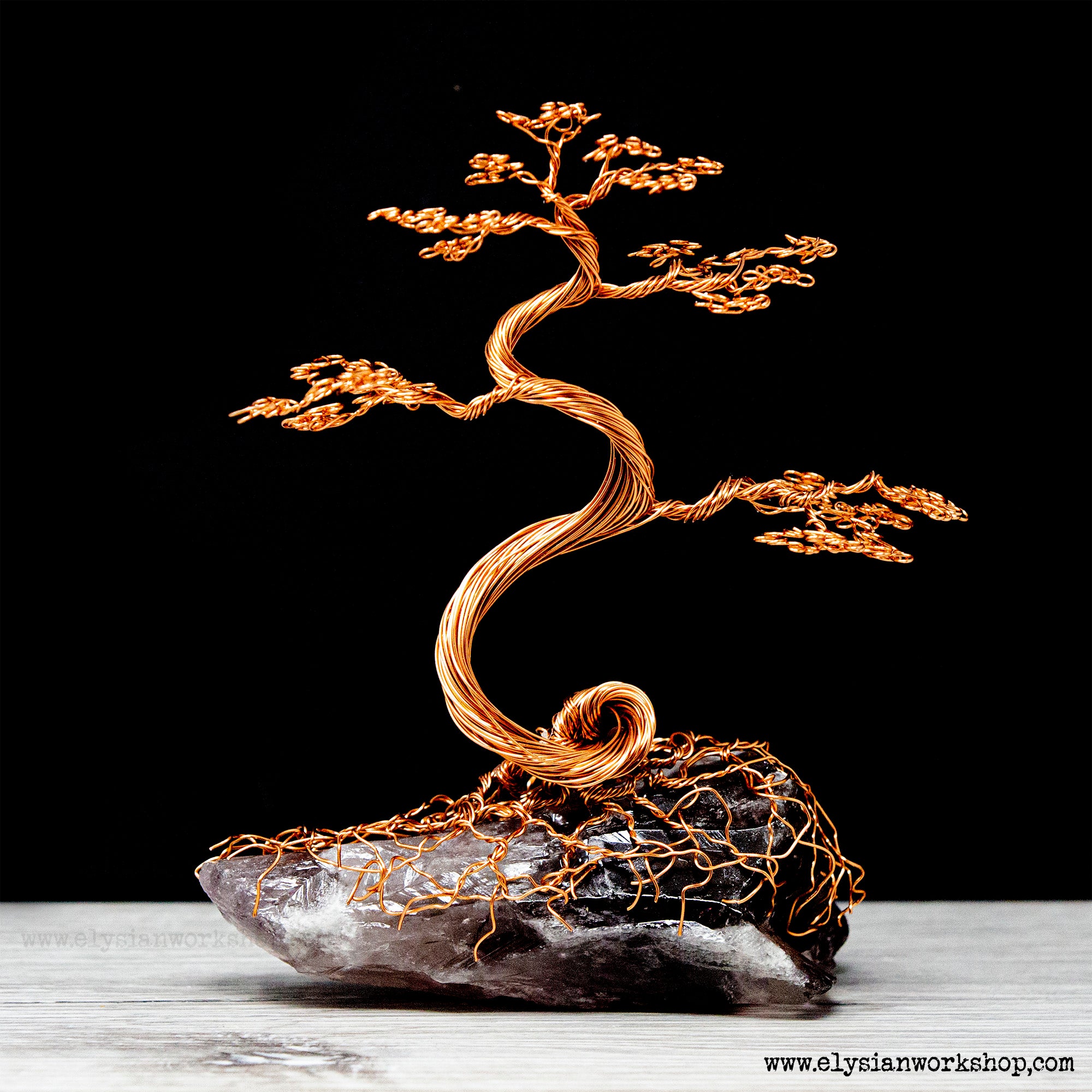This highly detailed studio photograph captures a stunning wire-twisting sculpture that resembles a bonsai tree. The tree is intricately crafted from strands of gold-colored wire, which form a main stalk that elegantly branches out into a series of delicate, wave-like branches. These branches extend to each side, creating a beautifully intricate structure. The base of the sculpture is anchored by a beautiful amethyst crystal, which is a captivating blend of purple and opaque hues. The tree’s base twists and loops around this crystal, forming a mesmerizing contrast between the metallic gold and the natural mineral.

The sculpture rests on a light gray, wooden-like surface, with a solid black background that enhances the visual prominence of the artwork. The photograph appears to be a professional studio shot, capturing the exquisite detail and craftsmanship of the piece. The web address "www.elysanworkshop.com" is subtly placed in black text at the bottom right corner of the image, without drawing attention away from the main subject.